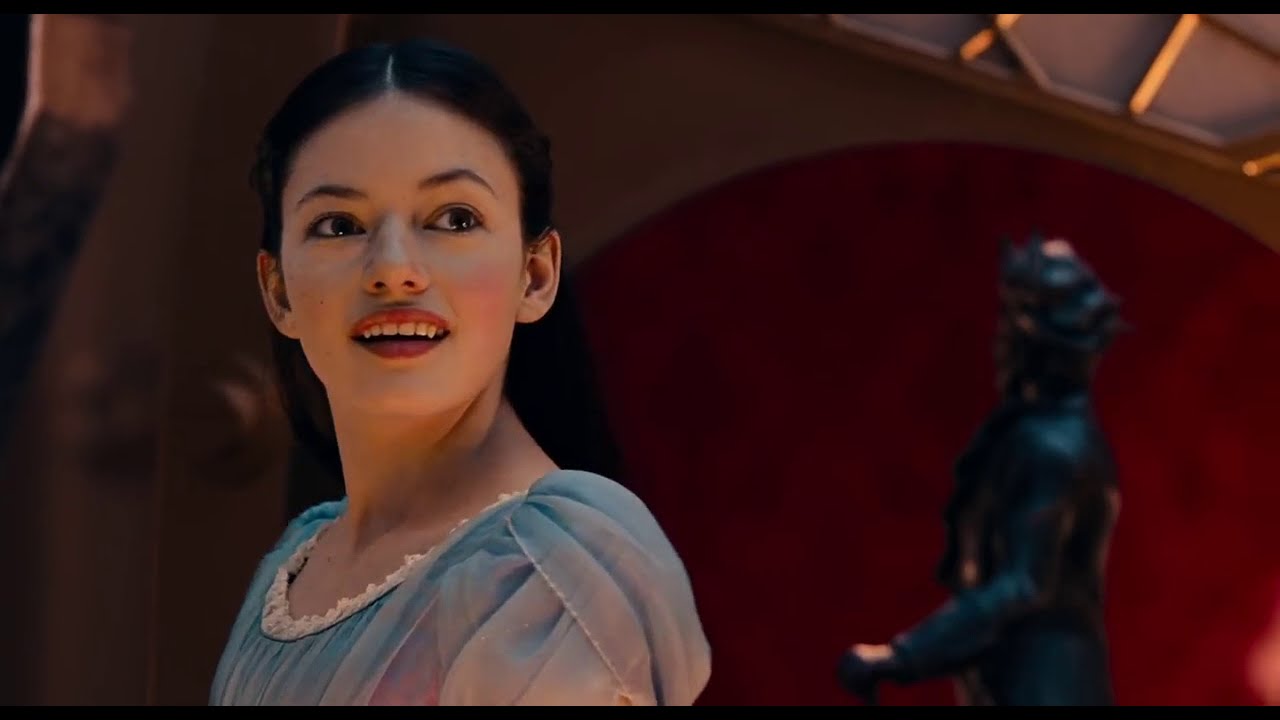The image depicts a scene from what appears to be a movie, featuring a young woman dressed in a blue, lacy dress with poofy shoulder pads. Her outfit includes a white lacy neckline. The woman, who has black hair parted down the middle and brown eyes, is slightly smiling with her mouth half-open, revealing her top teeth. Positioned towards the left of the frame, her body faces left while her head and gaze are turned towards the camera.

In the blurred background, to the right, stands a black statue of a human figure, which might be either a man or a woman holding something like a cane, and possibly adorned with a lot of hair or a hat. Behind the statue, the wall is marked by a large red circle, while the upper part of the wall features a gold or brown flat surface with intricate designs. Additionally, on the left side of the image, partially out of focus, there's a detail resembling a doorknob or a large button. The background elements, combined with the woman's poised look, hint at a scripted, cinematic setting.